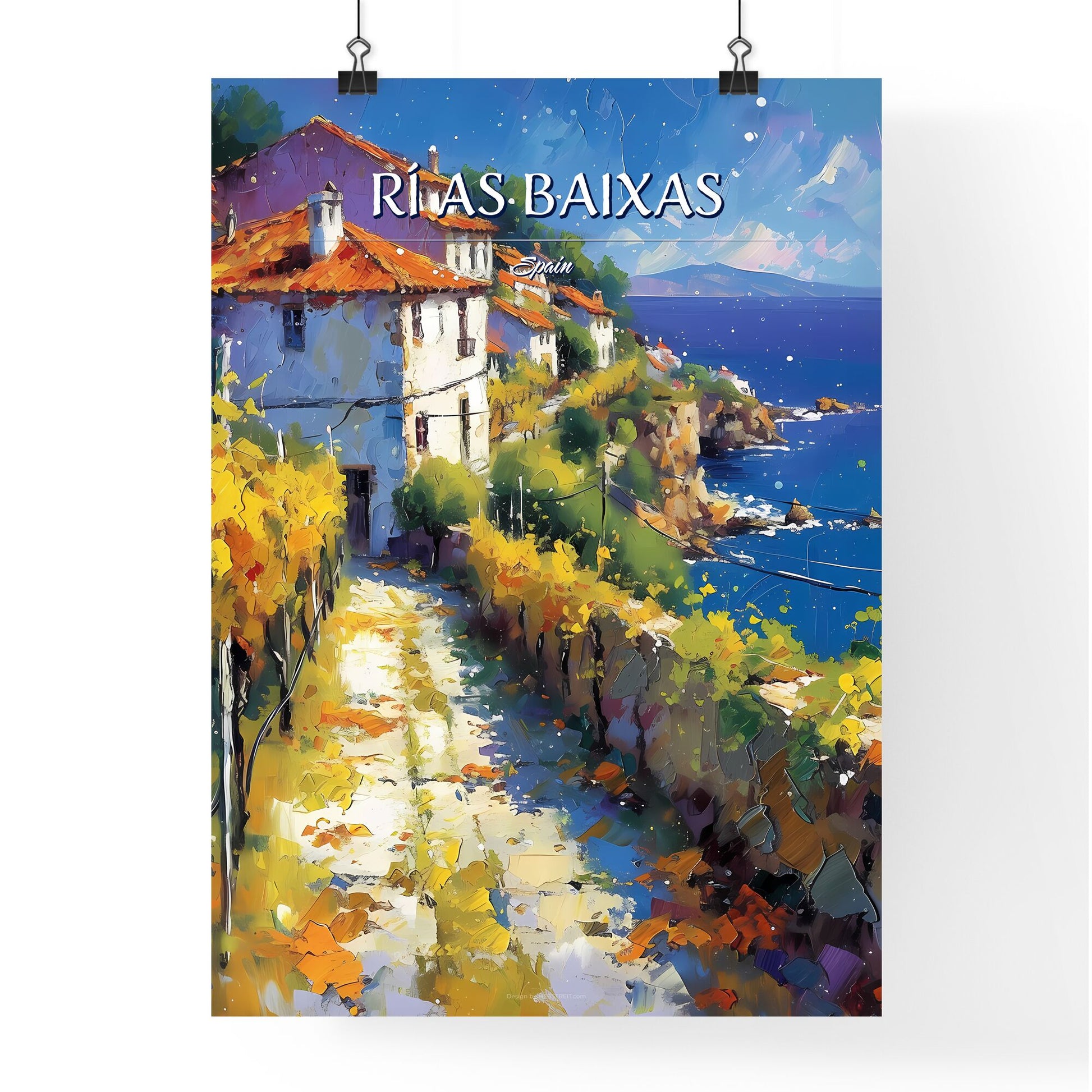This is an intricate painting displayed as a poster, held up by black metal clips. The image depicts a picturesque coastal village labeled "Rias Baixas, Spain." The scene unfolds with a white pathway flanked by lush foliage, leading towards a prominent white house with a tan roof, possibly made of Spanish tile, featuring a chimney. The village, made of stone, showcases moss and grass growing along the stone walls. In the background, similar quaint houses and a blue-gray mountain can be seen, with the right side of the painting revealing a waterway lined with more foliage. The tranquil blue waters and white clouds further enhance the beauty of this Spanish seaside village.